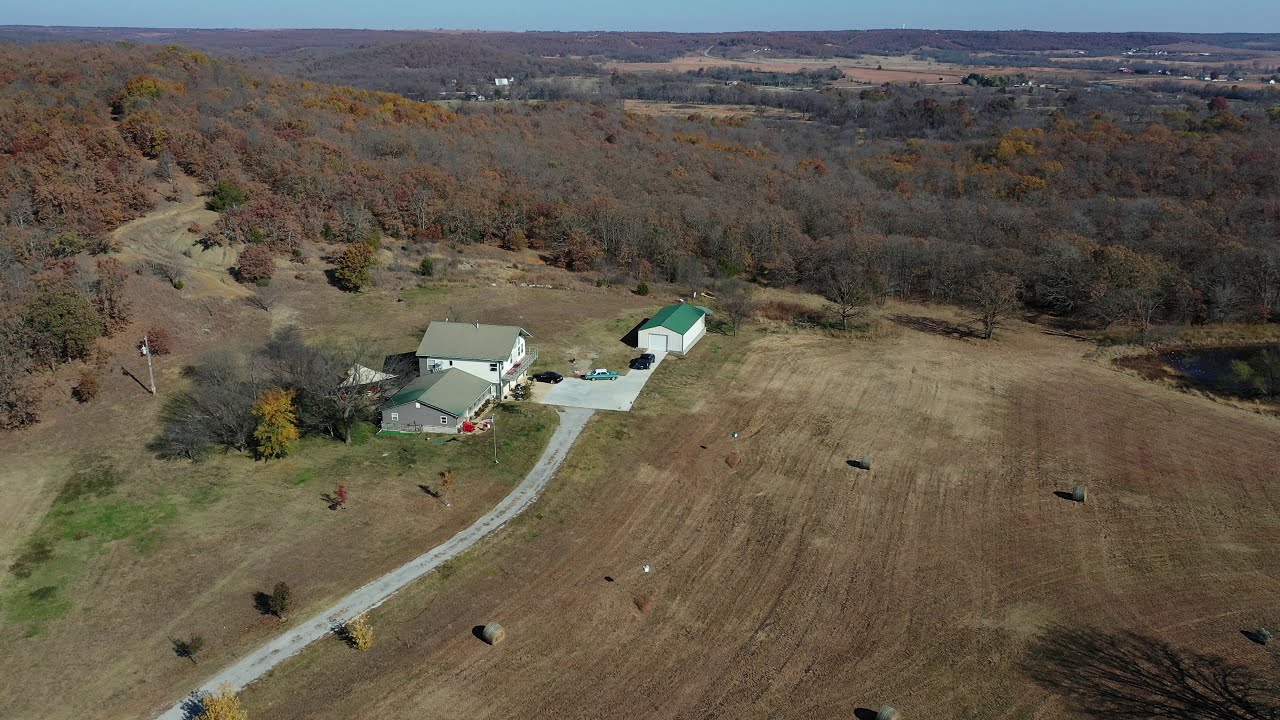The photograph captures an expansive rural landscape from an aerial viewpoint, showcasing a large, predominantly brown field marked with tire tracks and rolled hay bales. To the left, a narrow strip of green grass flanks a long paved driveway that leads to a house with a distinctive architectural style. The house features a taller, two-story white section with a front porch, connected to a lower, one-story gray extension. In front of the house, a paved parking area accommodates a black car, a turquoise car, and another vintage vehicle.

Adjacent to the parking lot is a long, white building with a green roof, which could be a garage or shed. Behind and to the left of the house stretches more open field, culminating in a forest of vibrant fall foliage, with colors ranging from dark red to orange and hints of gray. The backdrop includes a slight hill that leads up to the forest, which then continues into the distance. Far beyond, additional fields and patches of woodland are visible, alongside a few scattered farm buildings in clearings, especially in the top right and left portions of the image. The scene is bathed in natural daylight, highlighting the vastness and variety of colors within the landscape.